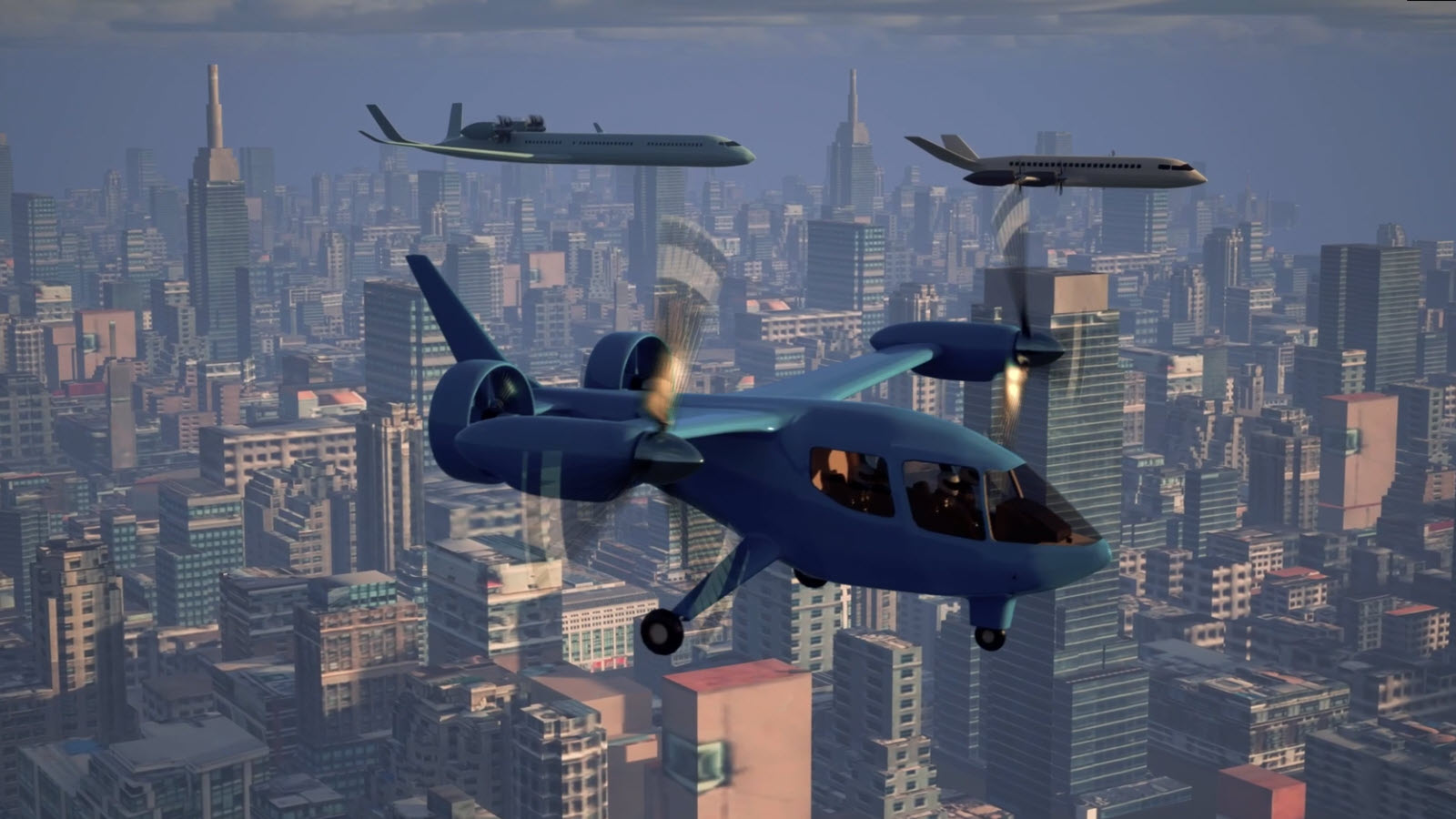In an aerial view, a drawing captures the dynamic scene of a futuristic city shrouded in a smoky, foggy haze, reminiscent of New York at sunset. Dominating the sky are three distinct aircraft. At the forefront, a royal blue, small helicopter-like plane hovers, notable for its hybrid design featuring wings with propellers and two large round fans flanking its tail. This advanced craft rests on three landing wheels and boasts a cockpit with five large, slightly bent windows where a sunglass-wearing pilot is visible. 

Trailing behind are two jets—one white and the other either gray or light blue—with sleek, modern designs deviating from contemporary airplane aesthetics. These jets, larger than the blue craft, appear to be passenger airplanes, with the one closer to the right side being smaller than the one on the left. The entire scene, seemingly lifted from a video game or artist's rendition, unfolds from an elevated perspective, capturing the futuristic cityscape below under an overcast, gray sky.